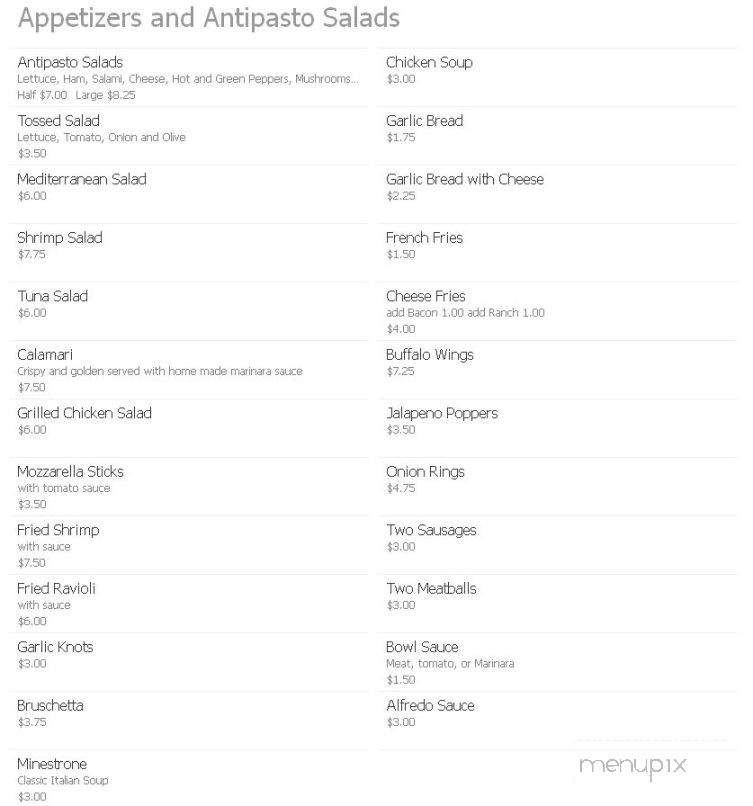**Menu: Appetizers and Antipasto Salads**

**Antipasto Salads:**
- **Antipasto Salad:** Lettuce, ham, salami, cheese, hot and green peppers, and mushrooms. Available in half or large sizes.
- **Tossed Salad:** Lettuce, tomato, onion, and olives.
- **Mediterranean Salad:** Priced at $6.
- **Shrimp Salad**
- **Tuna Salad**

**Seafood and Additional Options:**
- **Calamari:** Described as crispy and golden, served with homemade marinara sauce.
- **Grilled Chicken Sandwich:** Priced at $6.
- **Mozzarella Sticks:** Served with tomato sauce, priced at $3.50.
- **Fried Ravioli**
- **Garlic Knots**
- **Bruschetta**

**Soups:**
- **Minestrone Soup (left column)**
- **Chicken Soup (right column)**

**Sides and Add-Ons:**
- **Garlic Bread**
- **Garlic Bread with Cheese**
- **French Fries**
- **Cheese Fries:** Option to add bacon or ranch for an additional $1.
- **Buffalo Wings**
- **Jalapeno Poppers**
- **Onion Rings**
- **Two Sausages**
- **Two Meatballs**
- **Bowl of Sauce**
- **Alfredo Sauce**